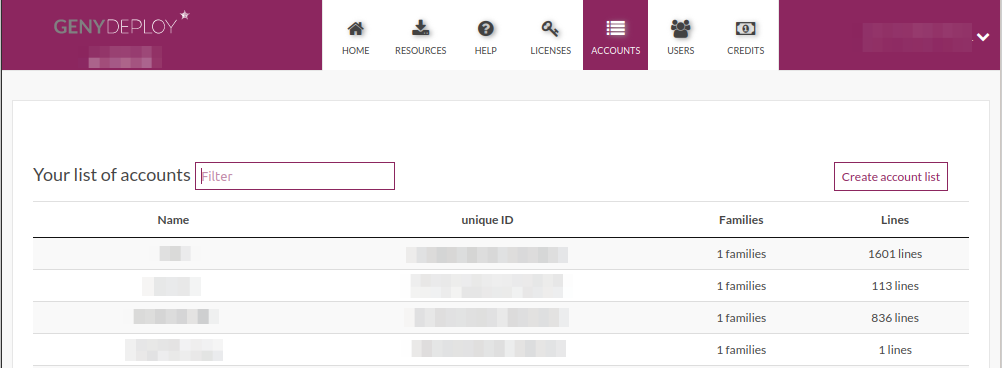The image depicts a digital interface with a structured and visually distinct layout. At the top of the interface, a burgundy banner spans the width of the screen. Positioned towards the right side of the banner, the text "GENY" is displayed in bold, green capital letters, followed by "DEPLOY" in a thin, white capital font. On the top right corner, there's a white star or asterisk symbol. Beneath this, a section with white text is present but appears pixelated and unreadable.

Moving to the center of the image, a vertical menu against a white background features several grey icons, each with corresponding labels in capital letters and shaded grey shadows beneath them. The icons are listed as follows from top to bottom:
1. A home icon labeled "HOME."
2. A download symbol labeled "RESOURCES."
3. A grey circle with a white question mark, labeled "HELP."
4. A grey key icon, tilted with the head towards the upper left and the key's bottom towards the lower right, labeled "LICENSES."

The fifth menu option is distinct, indicated as selected with a burgundy background and white icon and text. The icon consists of four horizontal lines with four dots to the left of each line, labeled "ACCOUNTS." Subsequent options revert to the grey and white color scheme:
6. An icon of three user silhouettes labeled "USERS."
7. A money symbol icon labeled "CREDITS."

On the far right of the screen, set against the burgundy background, a white arrowhead points downwards, indicating a dropdown menu.

Below the vertical menu, a white square area houses a table. On the top left of this section, the grey text reads "YOUR LIST OF ACCOUNTS." Embedded within this area is a rectangular input field with a burgundy border, featuring a cursor on the left and the word "FILTER."

The overall interface design is clean and organized, providing clear navigation and functional elements, accentuated by the burgundy and grey color scheme.